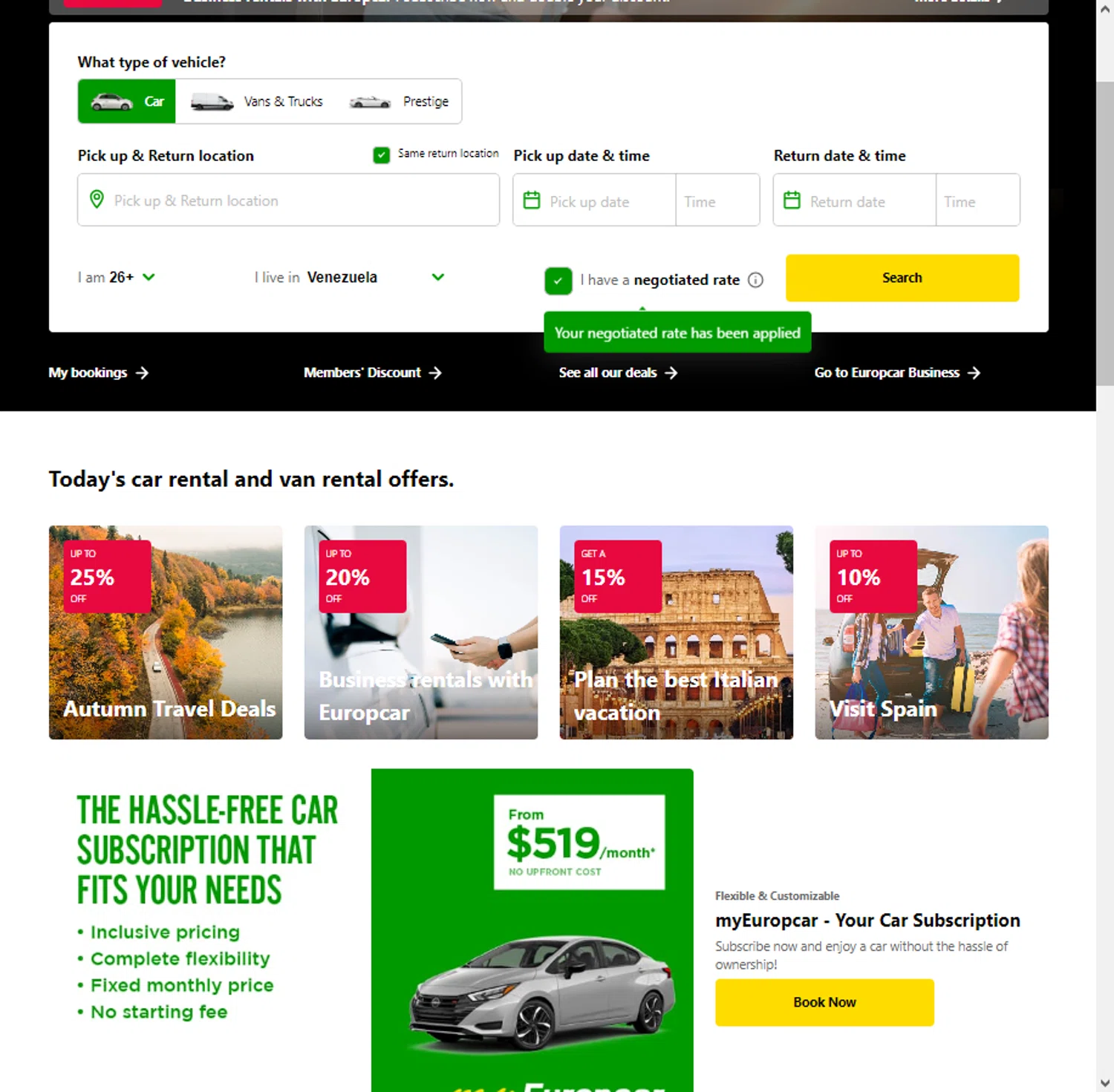The image displays a car rental booking interface set against a white background. The interface includes:

1. **Vehicle Selection**:
   - A green rectangle for selecting the type of vehicle, categorized into cars, vans and trucks, and prestige vehicles.

2. **Pickup and Return**:
   - Sections for specifying pickup and return locations, each with a search bar.

3. **Date and Time**:
   - Rectangles for entering the pickup date and time and the return date and time.

4. **User Details**:
   - An option indicating "I am 26+" with a checkbox, which is checked.
   - A field indicating "I live in Venezuela."
   - An option "I have a negotiated rate" with a checked checkbox.
   - A green rectangle that says "Your negotiated rate has been applied."

5. **Search Function**:
   - A yellow rectangle labeled "Search."

6. **Additional Options**:
   - Links to "My Bookings," "Members Discounts," "See All Our Deals," and "Go To European Business."

7. **Promotional Offers**:
   - A section titled "Today's Car Rental and Van Rentals Offers," featuring four promotional squares:
     - Up to 25% off Autumn Travel Deals
     - Up to 20% off Business Rentals with Europcar
     - 15% off planning the best Italian vacation
     - Up to 10% off visiting Spain

The overall interface is designed to facilitate easy navigation and selection of rental vehicles, dates, and locations while highlighting current promotional deals.